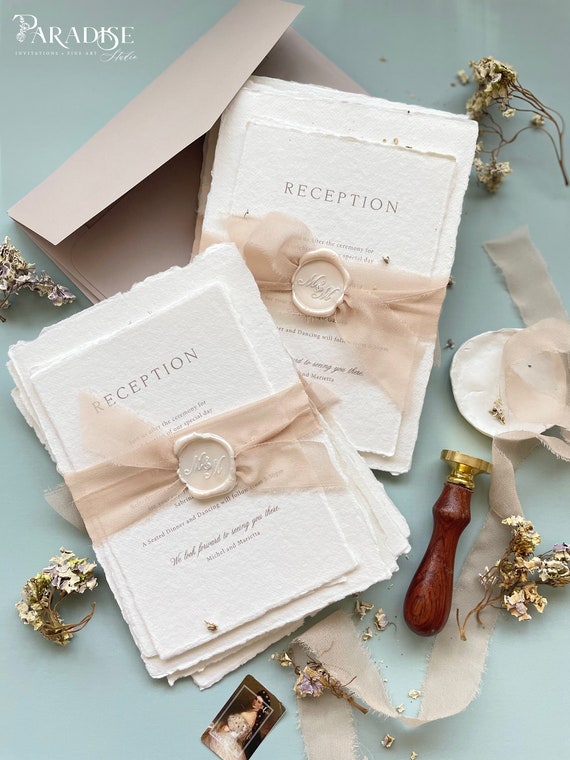This realistic photo features a meticulously arranged wedding reception invitation setup. Predominantly, you see two stacks of white invitations marked "reception", each tied with a piece of delicate taffeta ribbon featuring a seal. The stacks are slightly crossed over each other, resting on a beige envelope. In the top left corner of the image, the word "Paradise" is prominently displayed in white letters against a light teal-green background, with additional smaller text beneath it. Scattered across the table are sprigs of various plants and small florals. Near the center, there's a distinguished picture of a medieval woman in a wedding dress. Additionally, a wooden stamp with a gold end, presumably used for sealing the invitations, is placed among the other elements. The photo incorporates a palette of blue, white, pink, brown, green, and gray, contributing to its rich, inviting aesthetic.